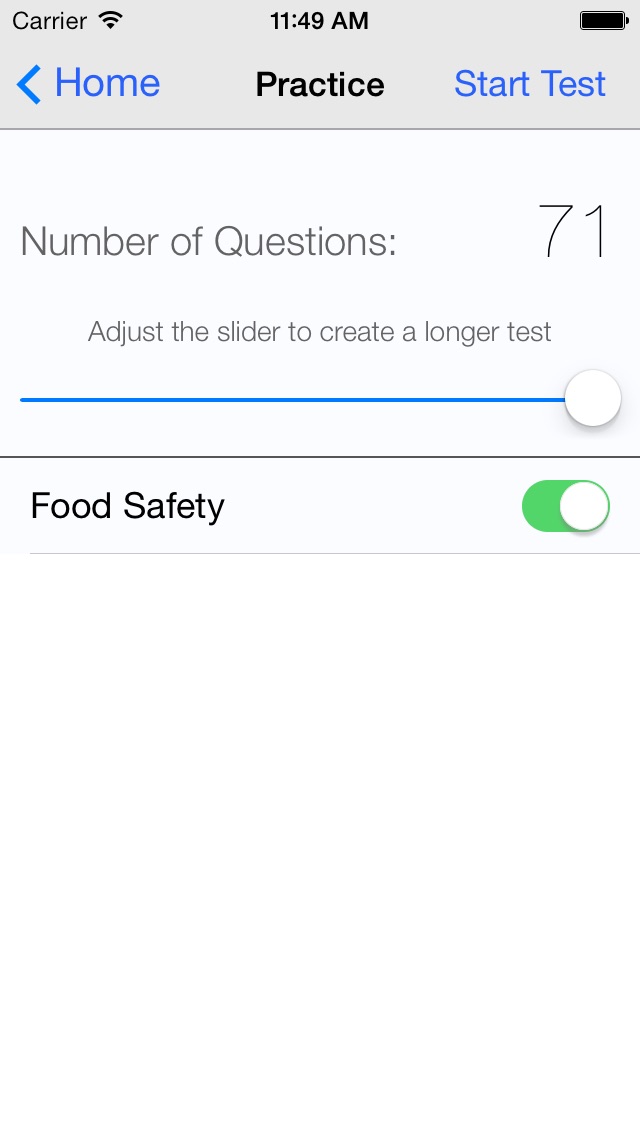The image displays a smartphone screen showing a detailed interface of a test preparation application. The status bar at the top indicates the time as 11:49 AM in black, with the carrier signal and a fully charged battery icon. The central part of the screen features three main sections: a "Home" button on the left, a "Practice" section in the center, and a "Start Test" button on the right, both highlighted in blue.

The "Practice" section currently displayed shows an option to practice test questions, indicating a total of 71 questions available. Users can adjust a slider to vary the number of questions for the practice session. Below this, there's a highlighted "Food Safety" category marked as enabled with a small green button, suggesting that users can enable or disable various categories for their practice sessions. Although only the Food Safety category is visible, it implies that other categories might also be available in the app.

Overall, this application appears to be designed to help users prepare for tests by customizing the number of practice questions and selecting specific categories, such as Food Safety.